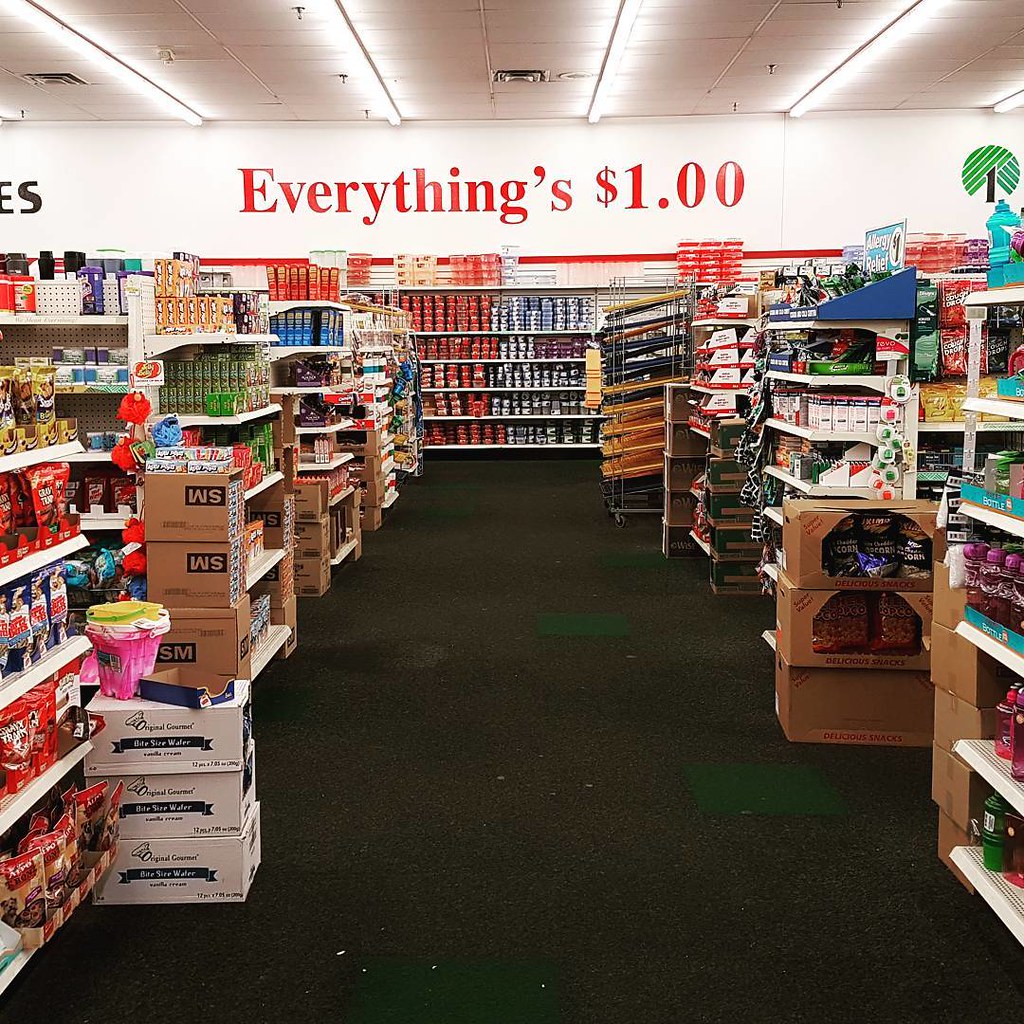The image captures the inside of a dollar store, presumably a Dollar Tree, as indicated by the recognizable tree logo with green grass at the top right of the image. Prominently displayed on the back wall is a large red sign that reads, "Everything's $1." The ceiling, painted in a white hue, features bright white lights arranged in vertical rectangular patterns, along with fire sprinklers. The store's black carpeted flooring stretches across the scene, surrounded by white shelves laden with a variety of colorful merchandise. Multiple aisles filled with different products are visible, indicating the extensive range of items available for just a dollar each.